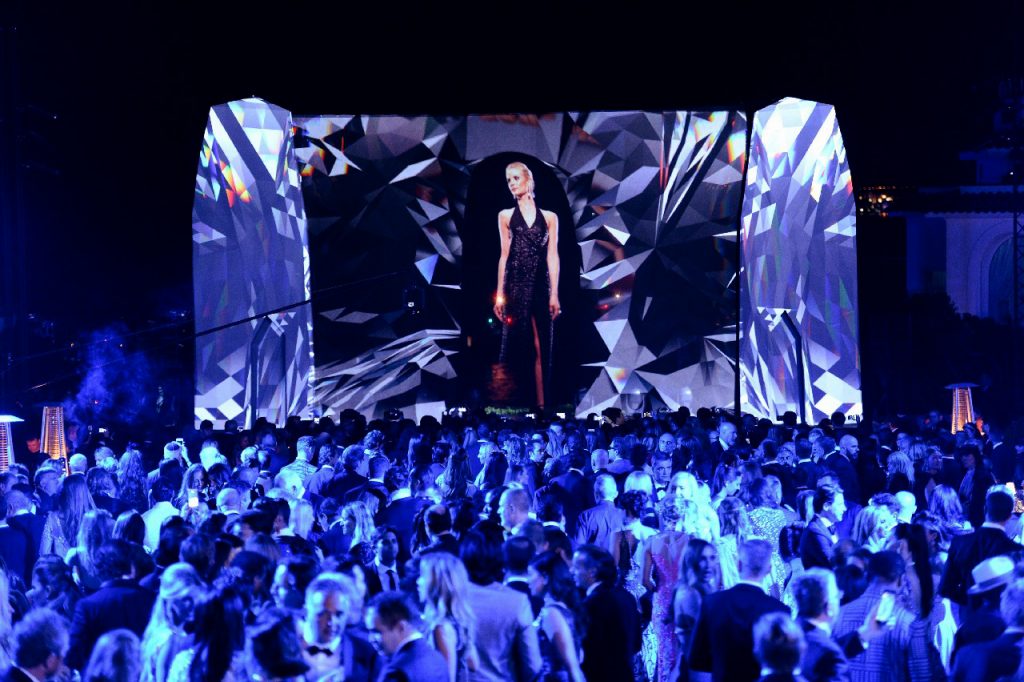The image depicts a nighttime outdoor event resembling an art show, concert, or formal party. Dominating the scene is a large, rectangular stage designed to appear as jagged, crystal-like formations that glow in blue hues against a pitch-black backdrop. Within these crystal formations is an exceptionally tall image of a woman with blonde hair, wearing a black gown that transitions into a burgundy rust color towards the bottom, suggesting that this image might be projected or computer-generated. Below the stage, a dense crowd of people dressed in formal black-tie attire—men in tuxedos and women in long dresses—mingle and converse, indicating that the performance or show has yet to begin.